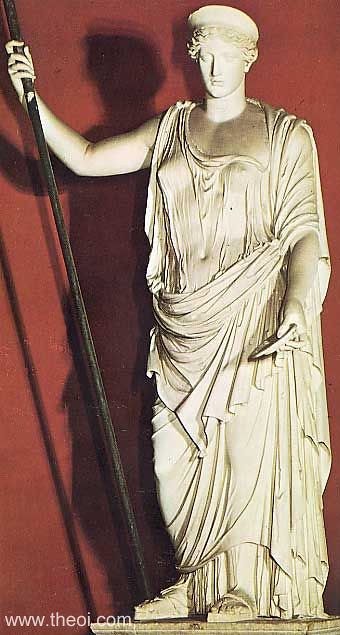This is a vertically aligned rectangular image of a classical statue set against a deep red wall. The statue, which appears to be made from a grayish-brown or silverish material, possibly marble, depicts a figure dressed in traditional attire resembling Roman clothing. The figure has its eyes closed, adding a serene expression to its face, and wears a hat over curly hair. Its right arm extends outward holding a dark brown or black pole, which could be a spear, while the left arm hangs by its side, grasping a small object, possibly a disc or plate. The draped robe features numerous ripples and reveals the figure's sandaled feet. A shadow of the statue and the pole is cast on the red wall behind it, indicating the direction of the lighting. In the lower left-hand corner of the image, the text "www.theoi.com" is visible. The statue stands on a square pedestal, though the full height of the pedestal is not shown in the picture.